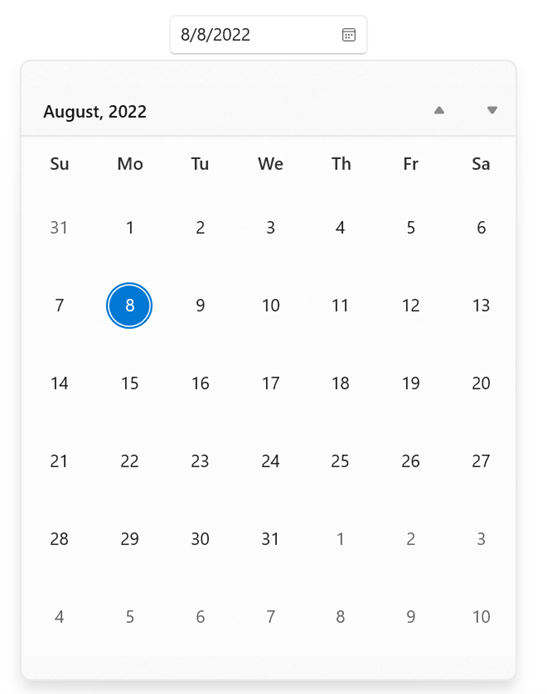The image depicts an open calendar application displaying the month of August 2022 in a layout reminiscent of a traditional printed calendar. The top section is highlighted with a gray border, and "August 2022" is clearly labeled in black lettering in the top-left corner. In the top-right corner, there are two gray triangles—one pointing up and the other pointing down—likely used for navigating between months. The calendar prominently features all 31 days of August, with additional visibility into 10 days of September and the last day of July, effectively showcasing parts of three months.

The layout shows that August starts on a Monday (the 1st) and ends on a Wednesday (the 31st). A blue dot marks August 8th, indicating it’s a highlighted date and also a Monday. Weekends are grouped and highlighted as follows: the 6th and 7th, the 13th and 14th, the 20th and 21st, and the 27th and 28th. This structured presentation helps users get a detailed overview of the month's schedule at a glance.